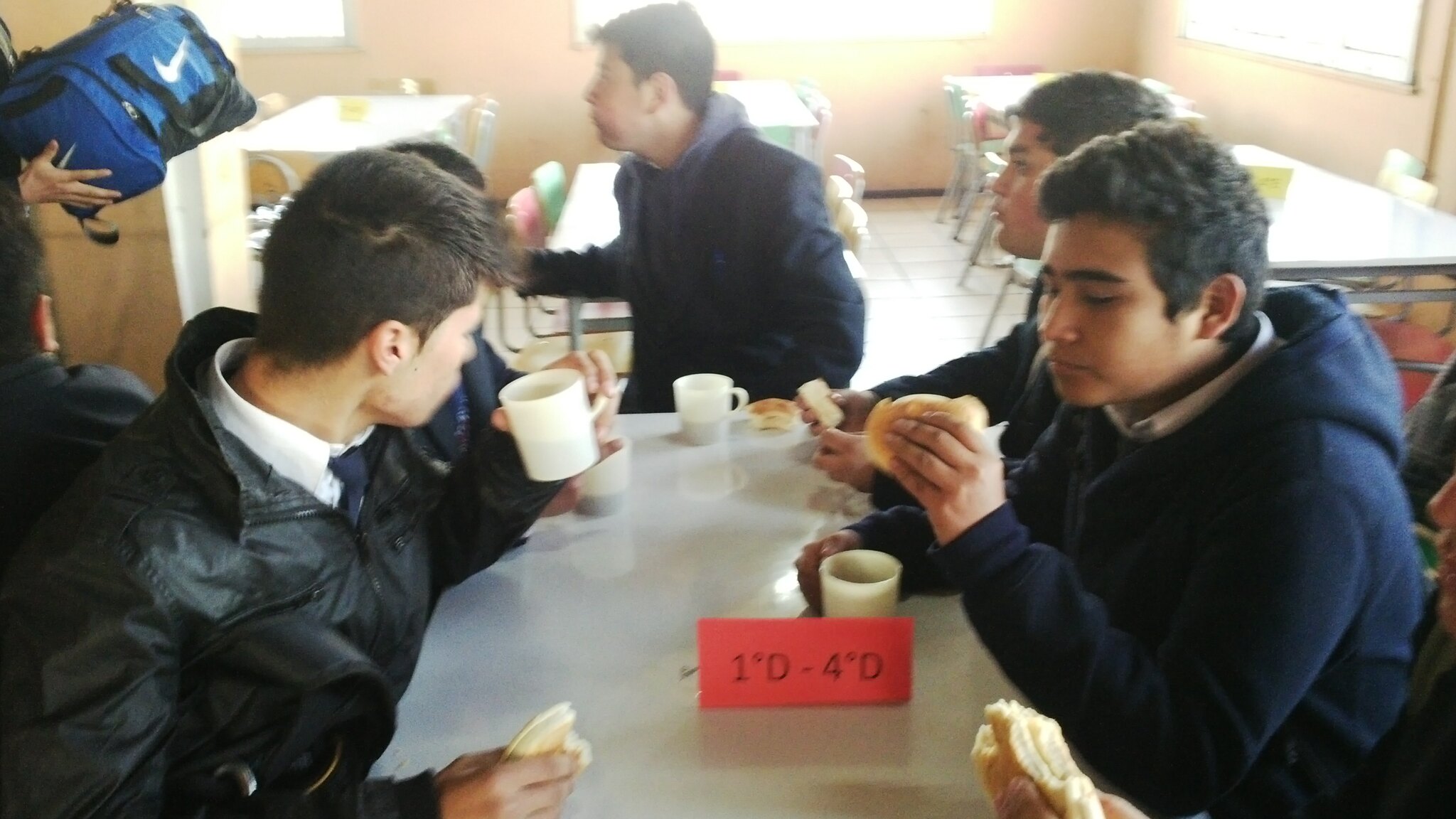This photograph features six teenage boys with similar dark brown haircuts and brownish to light brown skin. They are seated at a white table in what appears to be a school cafeteria, evidenced by multiple tables arranged for group seating. Each boy is dressed in a uniform consisting of a white collared shirt and a blue tie, with some also wearing jackets, suggesting it might be fall. They are drinking from white mugs and eating sandwiches or bread. A noticeable detail on the table is a red piece of paper labeled "1D-4D." In the upper left corner of the image, another person is partially visible, carrying a blue and black duffel bag, and interacting with one of the boys at the table. The overall setting resembles a dining room.